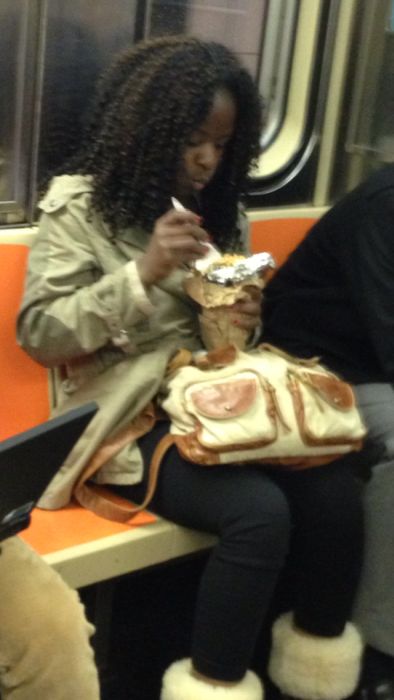In this detailed color photograph, an African-American woman is seated on a subway train, centrally positioned in the image. The subway bench she sits on is predominantly orange with white edges. She is wearing a grayish-green jacket over a beige top, black leggings, and black boots with white fluffy collars. Her long black curly hair cascades down as she looks attentively at the food in her hands. With a fork in her right hand, she is eating out of a piece of foil that rests in a paper bag held by her left hand. On her lap, there is a beige and brown handbag, its strap draped casually to the side. Behind her, the subway windows are visible, adding context to the scene. To her right, a man is partially visible, dressed in a black long-sleeve jacket and gray pants. In the bottom left corner, the knee of another person wearing beige pants is seen, along with the corner of an open laptop. The overall color palette includes black, brown, yellow, white, tan, and orange, accentuating the everyday urban setting.